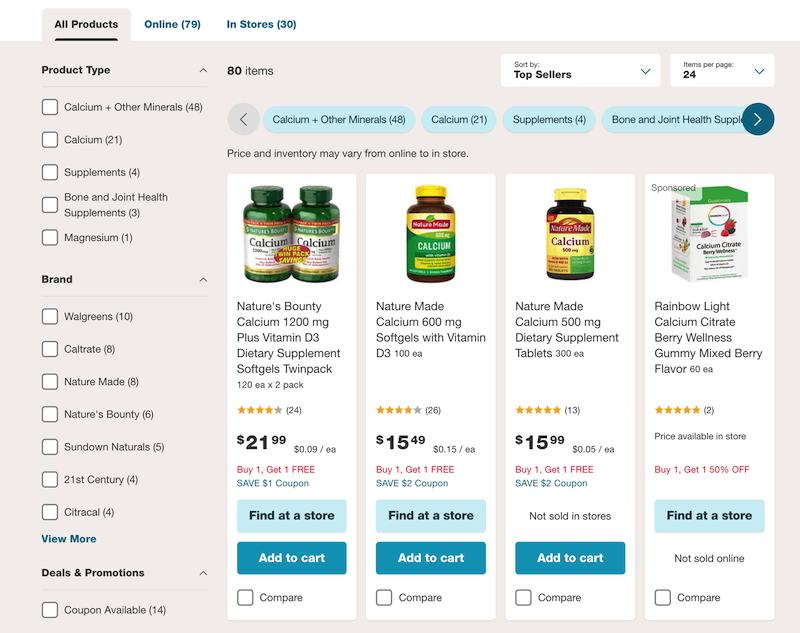**Detailed Caption:**

The screenshot showcases a landscape-oriented page from a supplement e-commerce site, likely Walgreens, offering vitamins and other dietary supplements. The top section of the website features three tabs: "All Products (79)", "Online only (79)", and "In Stores (30)". The "All Products" tab is currently selected.

The main section displays four vertical columns, each featuring various supplements:

1. The first column highlights "Nature's Bounty Calcium 1200 mg plus Vitamin D3 Dietary Supplement Soft Gels, Twin Pack" priced at $21.99. It includes a "Buy One Get One Free" promotion, a "$1.00 Off" coupon, and options to "Find at Store" and "Add to Cart".
   
2. The second column displays "Nature Made Calcium 600 mg Soft Gels with Vitamin D3" for $15.49, also with a "Buy One Get One Free" offer and a "$2.00 Off" coupon. Similar buttons for "Find at Store" and "Add to Cart" are available.

3. The third column features "Nature Made Calcium 500 mg Dietary Supplement Tablets" at $15.99. This product offers the same "Buy One Get One Free" and "$2.00 Off" promotional options but is marked as "Not Sold in Stores", with an "Add to Cart" button included.

4. The fourth column is marked as sponsored and presents "Rainbow Light Calcium Citrate Berry Wellness Gummies, Mixed Berry Flavor". This product comes in a box, unlike the others that are in bottles. Its price is only available in-store with a "Buy One Get One 50% Off" deal and a "Find at Store" button. It is not sold online.

The text for the promotions ("Buy One Get One" deals) is highlighted in red, whereas the rest of the text is mostly in black. Yellow star ratings are visible below each product, indicating customer reviews.

To the left of the product columns, there is a sidebar providing filter options categorized into "Product Type" and "Brand". Users can select from various product types such as magnesium, bone and joint health, and calcium supplements. Brand options include Walgreens, Caltrate, Nature Made, Nature's Bounty, Sundown Naturals, 21st Century, and Citracal. This additional detail suggests that the webpage is part of the Walgreens online store.

Overall, the layout is user-friendly, offering easy navigation through product categories and brands, ensuring a seamless shopping experience for supplements.